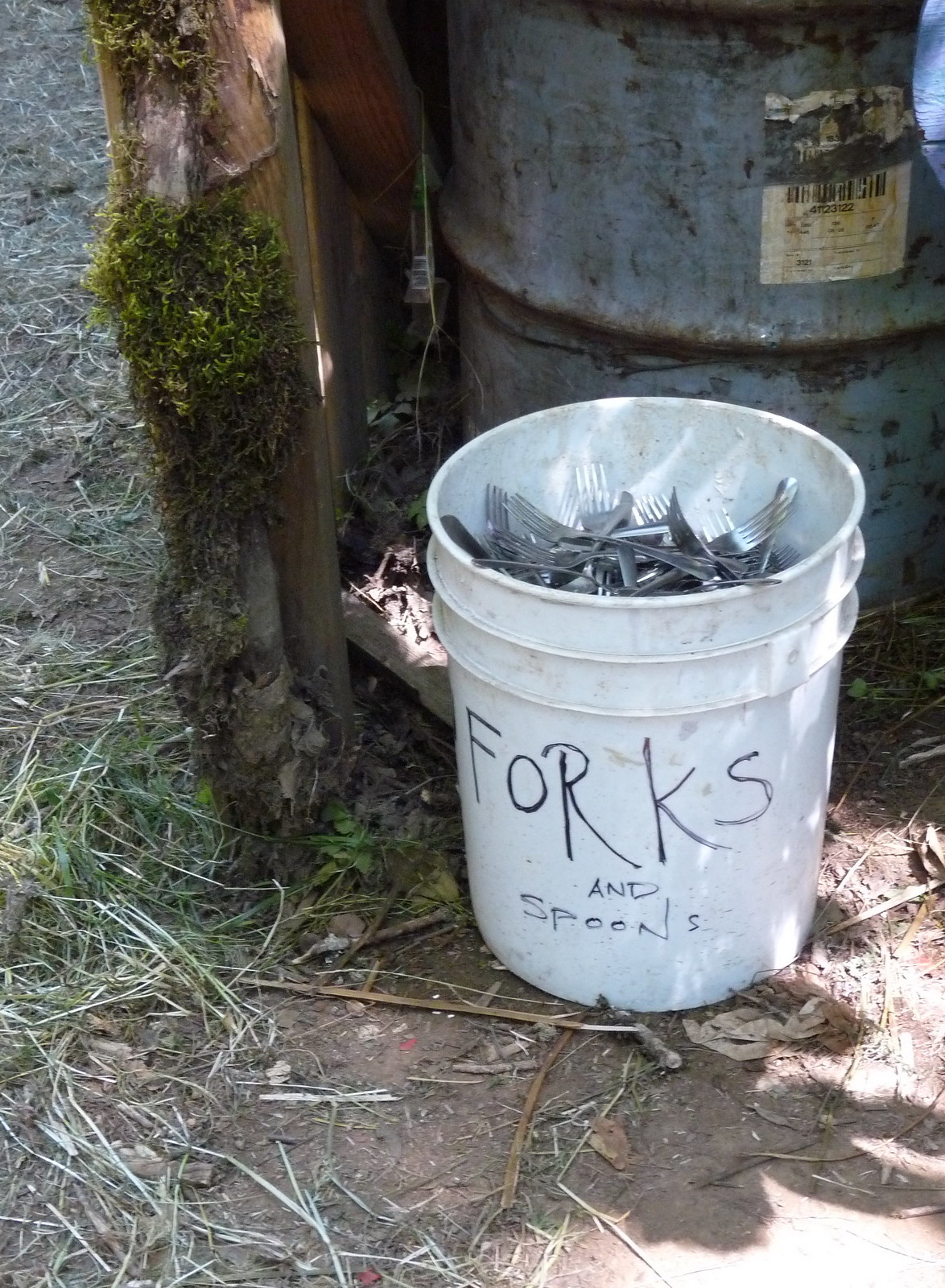In this outdoor photograph, the central focus is a dirty, white five-gallon bucket filled primarily with forks. The bucket is heavily soiled with smeared dirt marks and features a handwritten label in black marker that reads "Forks" in large, capital letters, followed by "and spoons" in smaller, smaller text. The bucket is three-quarters full and positioned on a mix of dirt, hay, and leaf litter, with thinly spread grass protruding. In the upper right-hand corner, a rusted 50-gallon steel drum, partially obscured from view, bears a tattered barcode with partially visible numbers (41123122). To the left and behind the bucket, a small wooden wall overgrown with algae, fungi, and creeping vines creates the backdrop. Shadows from nearby leaves or trees cast across the scene, adding to the image's rustic, neglected atmosphere.